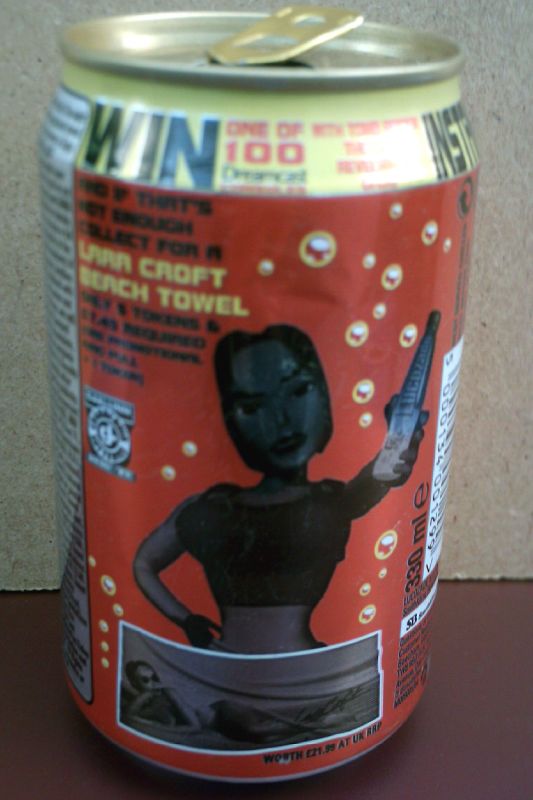The image features a red, 12-ounce soda can prominently displaying an advertisement for a contest. The can is decked with several vibrant visual elements and details. At the top of the can is a yellow-gold banner that announces a chance to "Win one of 100" prizes. Below this banner, the can showcases a striking cartoon image of Lara Croft, the iconic video game character, who is depicted with one hand on her hip and the other holding a bottle. The background behind Lara Croft consists of bubbles, adding a dynamic effect. To the left of her, there is text promoting a "Lara Croft beach towel," and above this, the word "Win" appears prominently. The can also displays "330 milliliters" on the right side, which is typical for a 12-ounce beverage can. There is an additional black-and-white image, possibly depicting a zombie, located below Lara Croft, adding a mysterious element to the design. The can is open at the top, revealing a small opening, and rests on a dark red table with a medium brown background. The entire can is brimming with vibrant advertisements and contest details, making it visually striking and information-rich.